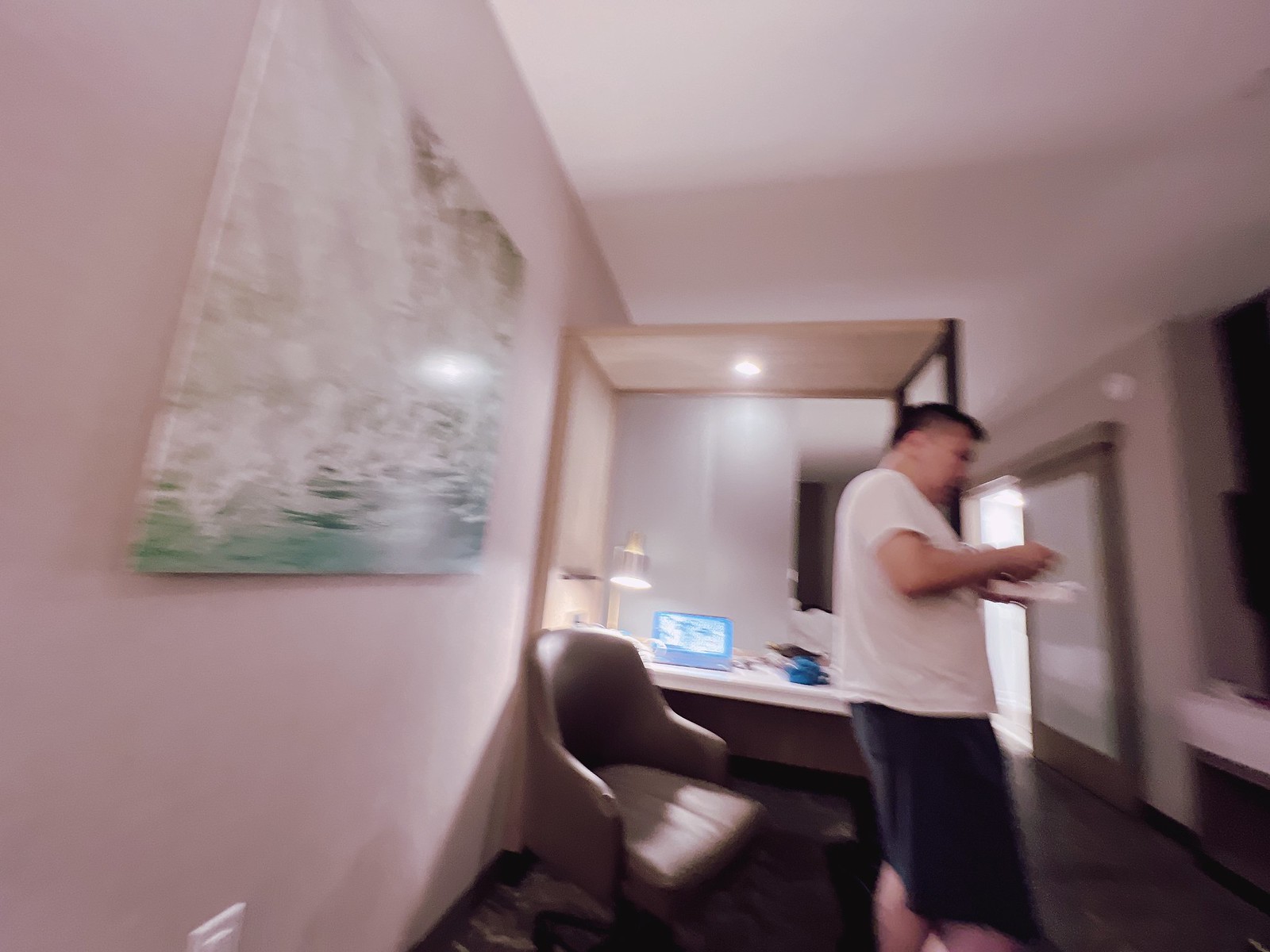In this slightly blurry photograph, a man with short dark hair is seen wearing a short-sleeve white shirt and darker-colored shorts. He holds a white food tray in his hands. In the background, a tan chair rests on a matching tan rug. An off-white wall serves as the backdrop, adorned with a painting featuring green, white, and gold tones. Adjacent to the chair, there is a desk made of light blonde wood with a white surface, hosting various items including an electronic device, a turned-on lamp, and blue and brown objects. A glimpse of the floor is visible, along with another wall that features a smoke detector and a door.